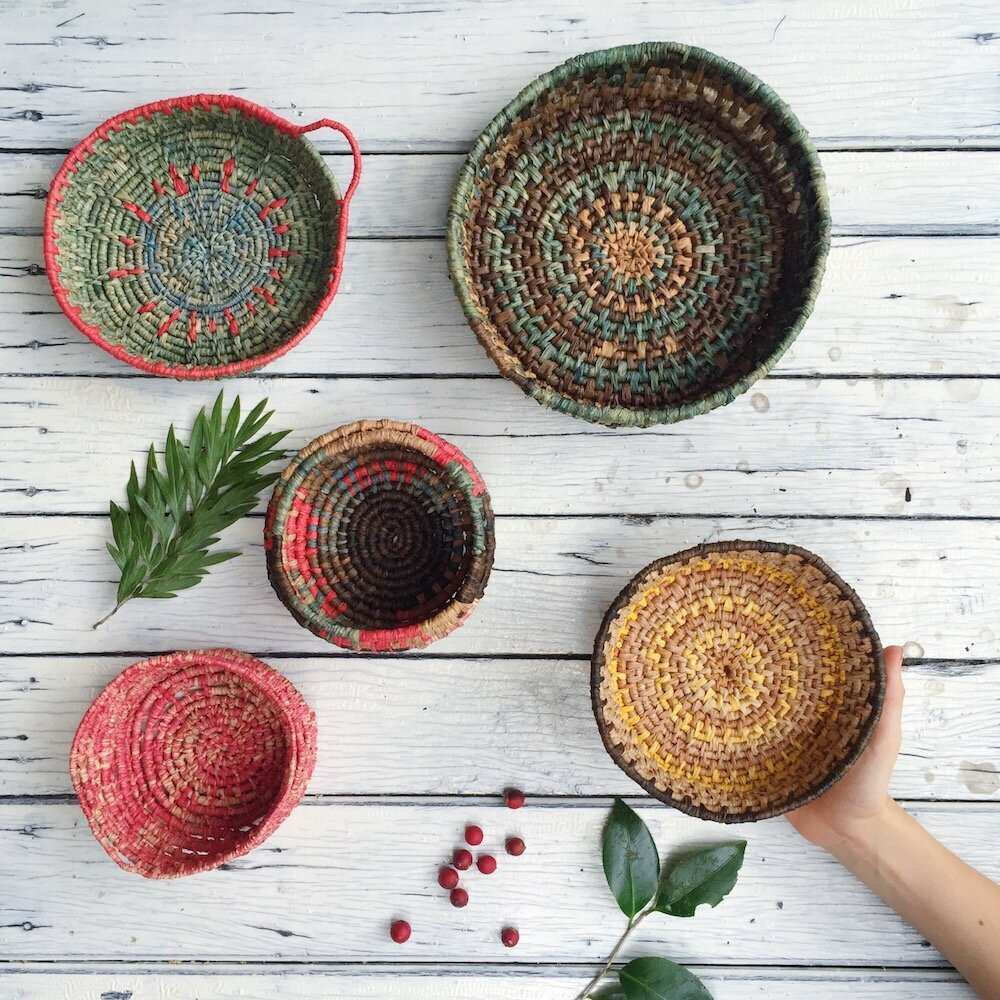This photograph captures a top-down view of five woven baskets, each varying in size and color, arranged on a horizontally placed wooden picnic table, painted with a shabby chic white finish. The baskets are diverse in their designs and textures. The top basket, medium-sized, features a red rim and a green interior. To its right, a basket showcases several concentric circles in shades of brown, green, and lighter brown at its center. Positioned centrally is one of the smaller baskets, resembling a cup with its red inside. Another small basket is on the lower left, noted for its flexibility due to thinner materials. The lower right basket, comparable in size to the top one, is being held by a person's right hand, illustrating the relative sizes. Scattered around the baskets are some green stems, possibly sprigs of rosemary, along with green leaves and several red berries.